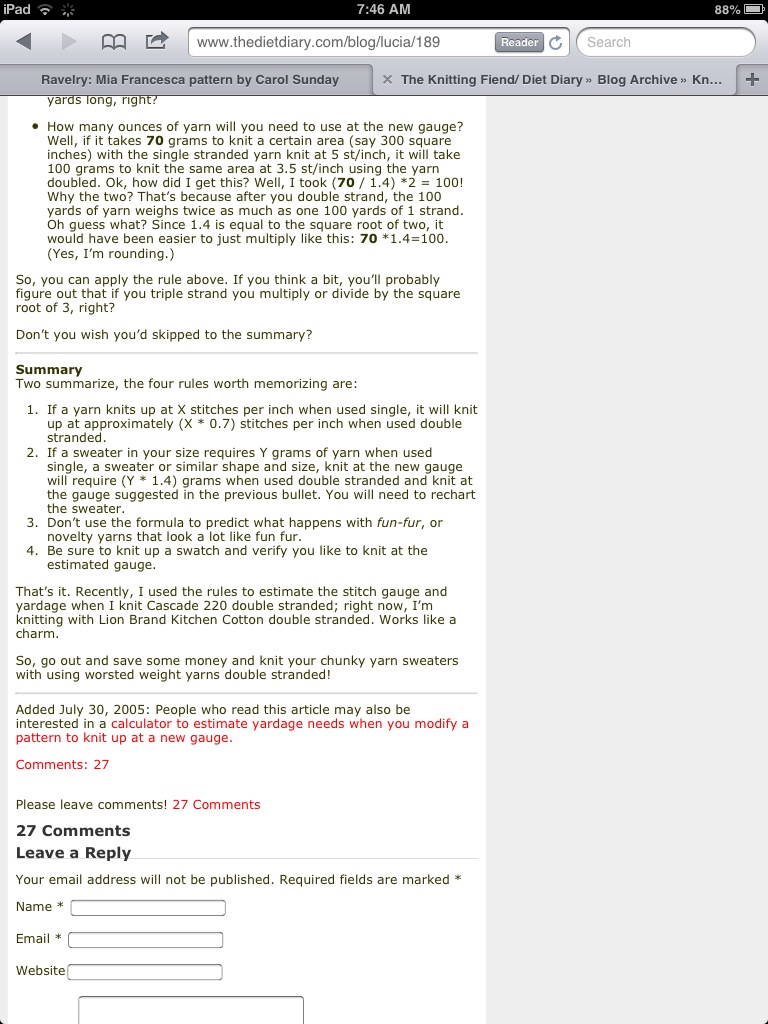This image captures a detailed screenshot taken on an iPad, showcasing a webpage filled with textual content. At the very top, the status bar displays "iPad" along with a Wifi icon indicating two signal bars, a spinning gear symbol, the time "7:46 AM" centered, and a battery status showing "88%" with a full battery icon. Below this, the URL bar reads "www.thedietdiary.com/blog/Lucia/189," with two open tabs: the left tab titled "Ravelry Mia Francesca pattern by Carol Sunday" and the right one "The Knitting Fiend / Diet Diary." Adjacent to the tabs are two squiggly arrow icons, indicating blog archive navigation.

The visible portion of the webpage features the conclusion of a blog entry concerning yarn usage calculations at different gauges. The text begins by explaining how to calculate the required ounces of yarn when changing the gauge, using a detailed example that transforms 70 grams of single-stranded yarn knitted at 5 stitches per inch into 100 grams of double-stranded yarn at 3.5 stitches per inch. This is followed by a mathematical breakdown and an explanation involving the square root of 2 for easier multiplication. The entry suggests a general rule for multi-stranding yarns and humorously advises readers to skip to the summary.

Below this, the blog provides a summary section, listing four memorization-worthy rules, followed by a concluding paragraph. The right third of the screen remains blank, while the left displays the textual content, formatted with paragraphs separated by horizontal lines. At the bottom, it prompts readers with "27 comments" and an invitation to "leave a reply," beside fields for name, email, and an unclear third input.